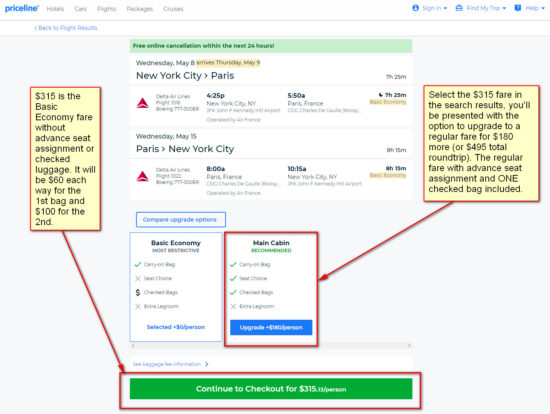This image is a detailed screenshot from Priceline.com, showcasing the flight booking options for a round trip between New York City and Paris. The layout is nearly square, suggesting it is likely from a computer rather than a cell phone. 

At the top of the screenshot, the Priceline logo is prominently displayed in blue. Below the logo, a light gray menu bar offers navigation options, including Hotels, Cars, Flights, Packages, and Cruises. In the upper right corner, darker blue font options for Sign In, Find My Trip, and Help are visible.

The primary content centers on flight details, illustrating a round trip from New York City to Paris, scheduled between May 8th and May 15th. Below the main flight information, there are two rectangular sections: one for basic economy and one for main cabin selection. The main cabin option is highlighted with a red outline, and a red arrow points to it from a nearby yellow-highlighted box with a red border, instructing users to "select the $315 fare in the search results" and providing additional guidance.

Further instructions continue below in another yellow-highlighted box with a red rectangular outline, connected by a red arrow to a green rectangle labeled "Continue to checkout for $315." The entire setup suggests that this image might be part of a tutorial or help screen designed to guide users through the booking process on Priceline.com.